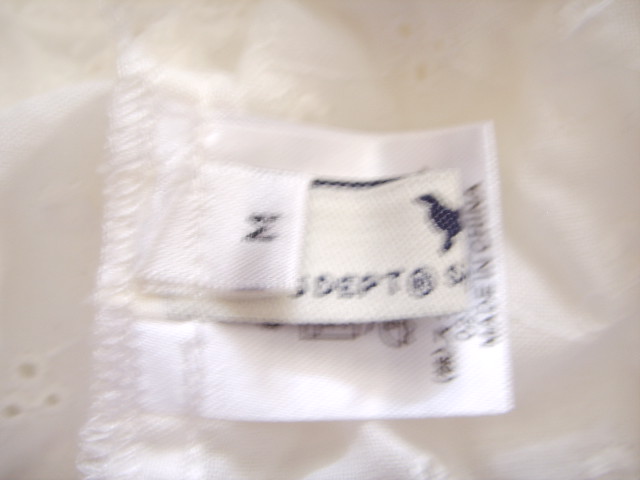A highly zoomed-in, blurry photograph features a piece of fabric, presumably a pair of women's panties or possibly a diaper. The image captures the waistband oriented to the left side of the frame. The waistband, along with the fabric, is white and rests on top of another white cloth. Focused prominently in the shot are three distinct white tags affixed to the waistband. The topmost tag is a small, square label displaying a bold black "M." Below it sits a longer rectangular tag with indecipherable text due to the blurriness. The third and largest tag, situated beneath the previous two, also contains unreadable writing because of the image's poor focus.